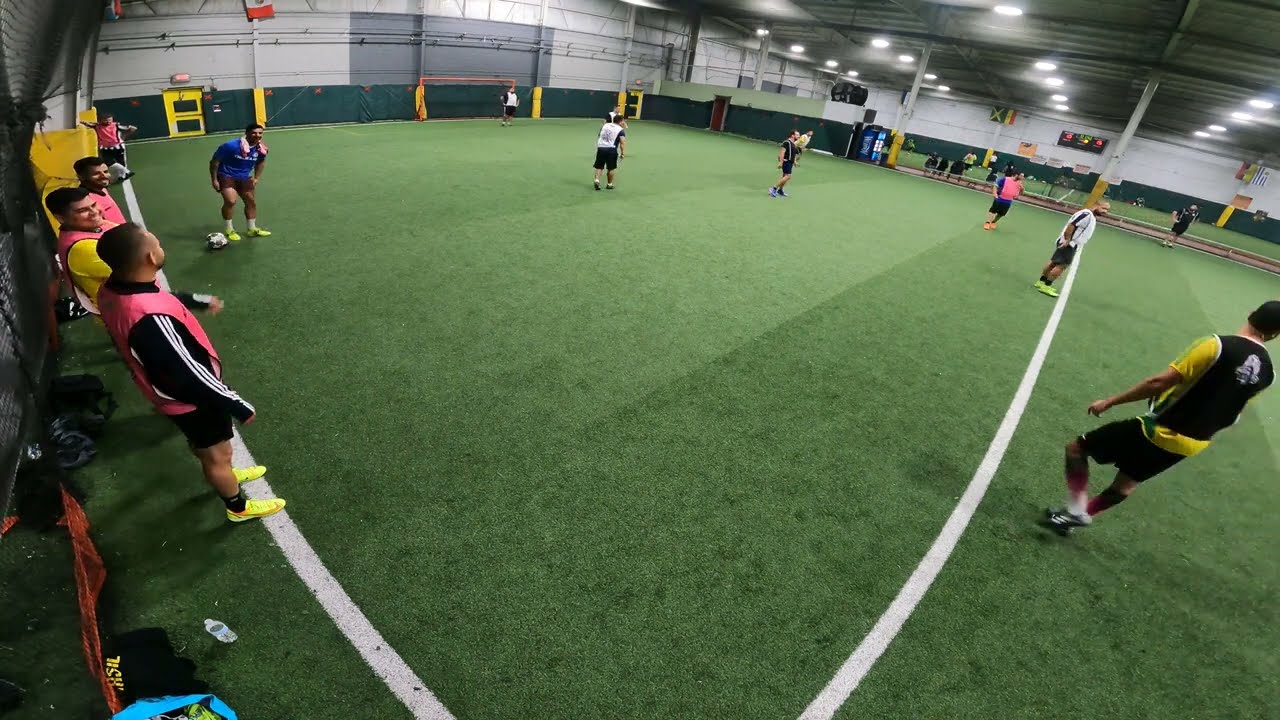This image depicts an indoor soccer practice set in a large, warehouse-like sports arena with multiple fields. The view captures an astroturf field, with various players positioned both on the sidelines and scattered across the middle of the field. On the left side of the image is a goal, and a goalie appears to be preparing to block an attempt. The players are divided into teams wearing distinct jerseys: one team in pink and the other in blue. Among them, one player stands out with bright yellow soccer shoes. A referee is also present on the field. The ceiling is equipped with numerous lights that illuminate the space, giving a clear view of the action despite the absence of natural light. The colors visible in the scene include green, blue, yellow, red, pink, grey, black, and white. No text is visible within the image.